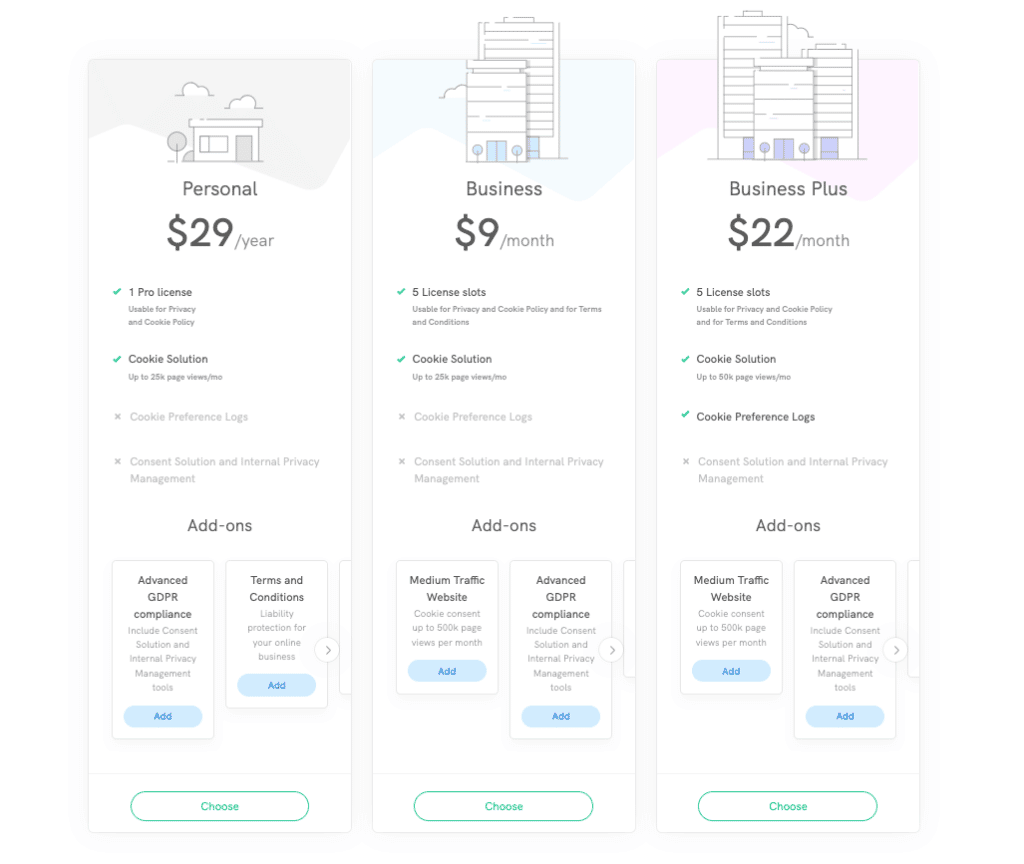The image showcases a subscription plan comparison set against a very light blue background. It features three vertically aligned boxes, each detailing a different plan.

**Box 1: Personal Plan ($29/year)**
- **Background Imagery**: Blue sky with clouds, a small house, and trees.
- **Features**:
  - **Pro License**: Blue check mark
  - **Cookie Solution**: Blue check mark
  - **Cookie Preference Logs**: X mark
  - **Consent Solution**: X mark
  - **Internal Privacy Pick Guard**: X mark
  - **Add-ons**:
    - Advanced GDPR Compliance: Blue "Add" button
  - **Terms and Conditions**: Blue "Add" button
- **Action Button**: White "Choose" button surrounded by blue

**Box 2: Business Plan ($9/month)**
- **Features**:
  - **License Slots**: 5
  - **Cookie Solution**: Blue check mark
  - **Cookie Preference Logs**: X mark
  - **Consent Solution**: X mark
  - **Advanced GDPR Compliance**: Blue "Add" button
- **Add-ons**:
  - Medium Traffic Website: Blue "Add" button
- **Action Button**: White "Choose" button surrounded by blue

**Box 3: Business Plus Plan ($22/month)**
- **Features**:
  - **License Slots**: 5
  - **Cookie Solution**: Blue check mark
  - **Cookie Preference Logs**: Blue check mark
  - **Consent Solution**: X mark
- **Add-ons**:
  - Medium Traffic Website: Blue "Add" button
  - Advanced GDPR Compliance: Blue "Add" button
- **Action Button**: White "Choose" button surrounded by blue

The detailed comparison helps users understand the different subscription offerings, clearly highlighting the available features, additional services, and pricing options.